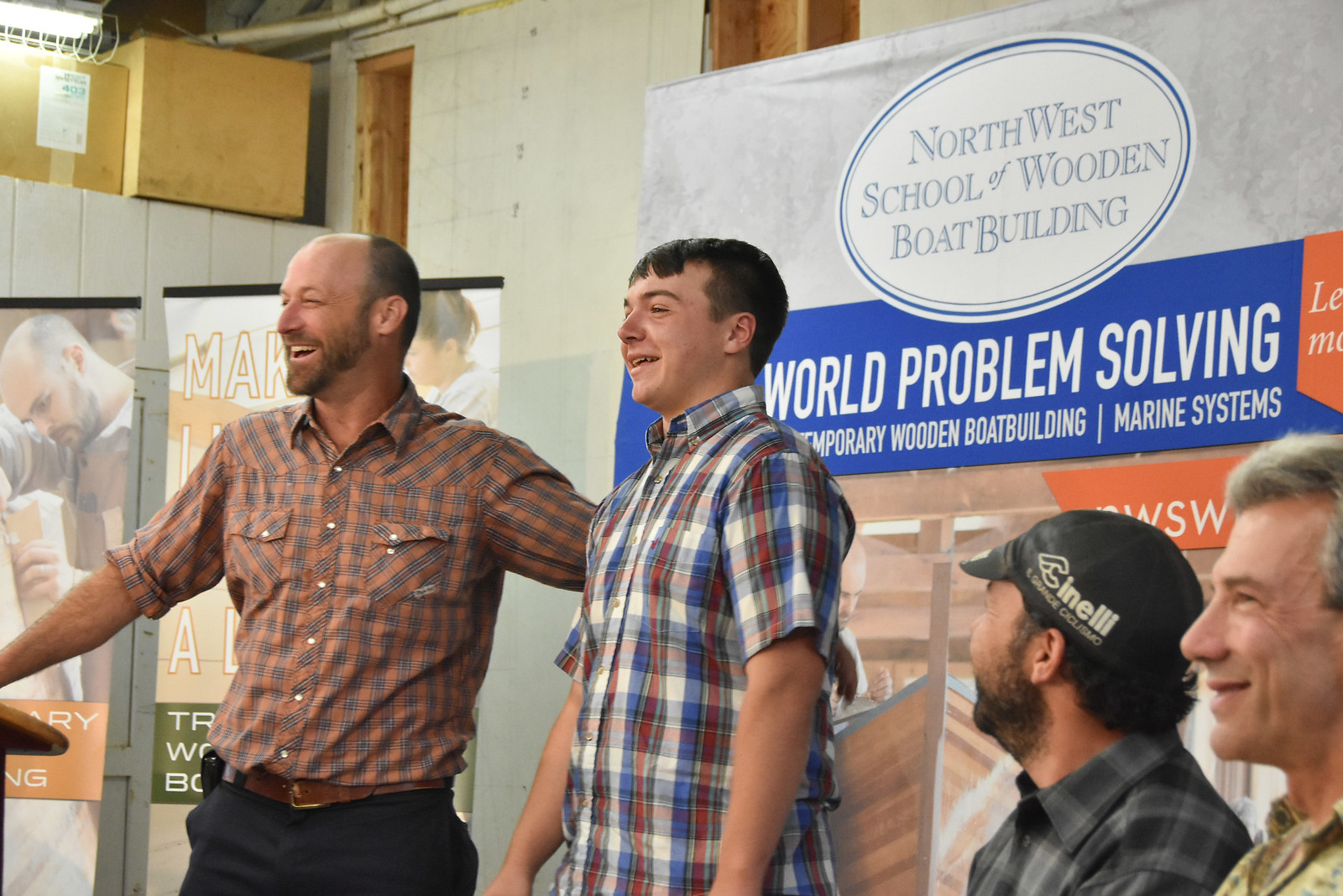The image depicts a lively scene of four individuals at an event associated with the Northwest School of Wooden Boat Building. The setting is brightly lit, suggesting strong sunlight filtering into the indoor venue. In the background, a prominent sign reads "Northwest School of Wooden Boat Building, World Problem Solving, Temporary Wooden Boat Building, Marine Systems," indicating a focus on maritime education and craftsmanship.

In the foreground, a bearded, bald man in blue slacks and a brown checkered shirt, with sleeves rolled up, stands at a speaking podium on the lower left corner of the image. His left arm rests on the back of a teenage boy, perhaps around 14 years old, who stands next to him. The boy, dressed in a short-sleeved checkered shirt and sporting a bowl cut, smiles brightly, hinting at a significant achievement, possibly having built his first boat.

Seated to the right are two men, dressed in flannel-like shirts typical of laborers or craftsmen. The third man from the left wears a cap with the word "CINELLI" or a similar lettering. These men, like their standing counterparts, share in the moment's joy, smiling and exuding a cheerful demeanor. The backdrop shows several pictures and boxes with numbers and lines, possibly displaying the school's projects or advertisements. The palette of colors in the image comprises blue, white, orange, brown, and black, enhancing the vibrant yet industrious atmosphere of the event.